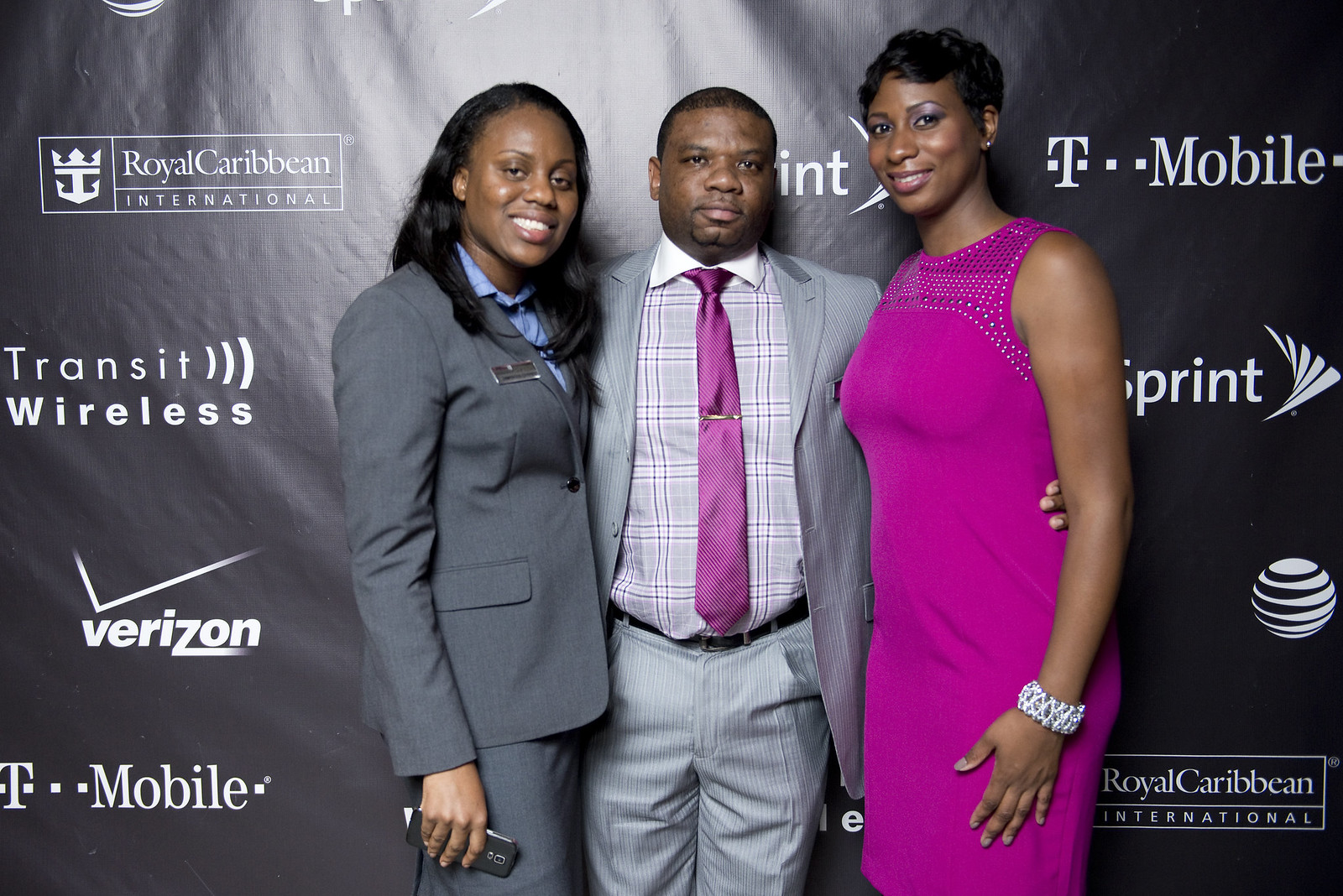This horizontally aligned rectangular color photograph captures three African American individuals posed on a stage. The backdrop features a large black banner with various sponsor logos, including Royal Caribbean International, Transit Wireless, Verizon, T-Mobile, and AT&T, prominently displayed in white text.

In the center stands a man in a light gray suit jacket and pants, paired with a purple tie and a checkered button-down shirt with a white collar. He has very short black hair and is looking directly at the camera without smiling. 

To his left, a woman dressed in a darker gray business suit and pants, with a blue button-down shirt underneath, is holding what appears to be a remote control in her right hand. She also sports a name tag on her right chest, though its details are unreadable. This woman has long black hair and is smiling at the camera.

On the man's right, another woman is wearing a purple sheath dress adorned with beads at the top and a large silver bracelet on her left wrist. She has short black hair and is also smiling warmly at the camera.

The photograph emphasizes a professional setting and the individuals’ business attire, framed by the backdrop of corporate logos.